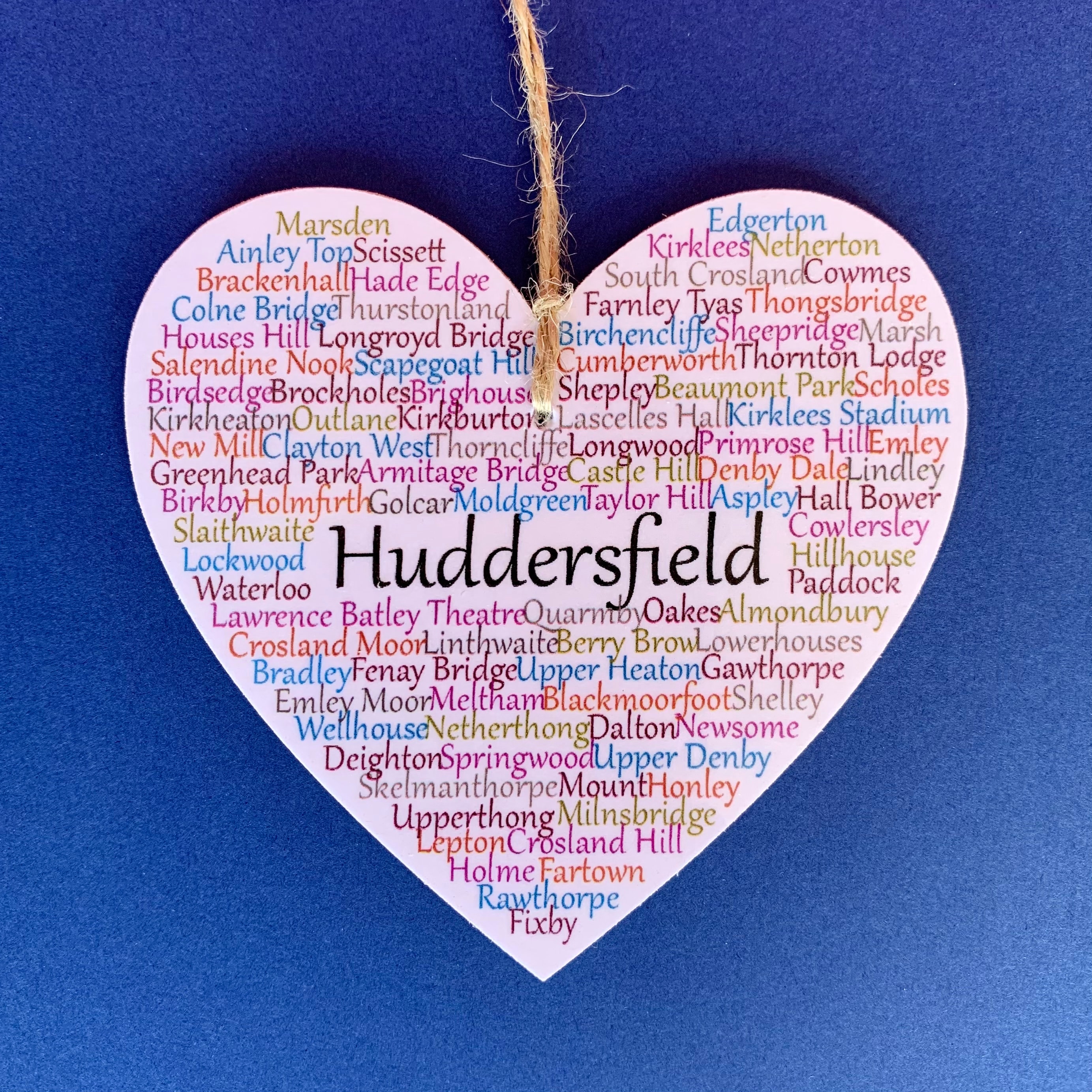This image is a captivating square photograph, six inches by six inches, with a plain blue, slightly blotchy background that resembles blue construction paper. At the top center of the image, a thin, furry rope descends and attaches to the top center of a large, light pink heart. This heart is covered in colorful text, featuring names of what seem to be locations. In bold black print at the center of the heart, the prominent word "Huddersfield" stands out, surrounded by names such as Marsden, Ainley Top, Edgerton, Kirklees, Netherton, South Crossland, Netherlong, Wellhouse, Dalton, Newsome, Upper Dong, Crossland Hill, Fixby, Brackenhall, Haydedge, Calmbridge, Thurstonland, and more. These names are written in various vivid colors including blue, orange, purple, red, gold, and pink, creating a vibrant mosaic of text across the heart. The heart, attached by the twine, seems ready to be hung, contributing to the overall whimsical and visually engaging composition.